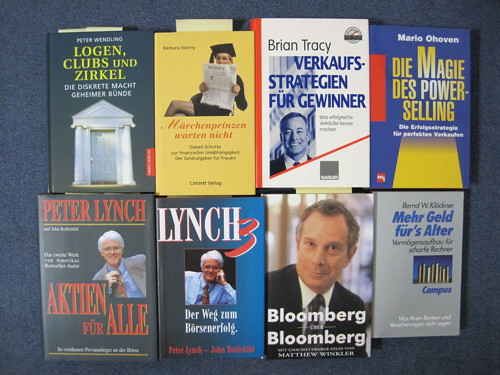This image is a slightly washed-out, color photograph taken with a flash, depicting eight books aligned in two columns of four. The books are laid out on a dark blue background, possibly a piece of paper or cardboard, and their edges touch each other. The books, mostly in German, feature a variety of covers in different colors: blue, red, yellow, dark gray, black, and silver. 

The bottom row includes two books by Peter Lynch, with one title partially visible as "Attica for Owl," and another titled "Lynch III." The book next to these, authored by Matthew Winkler, is titled "Bloomberg," featuring a man in a black suit and white shirt on the cover. The last book on the bottom row, by Bernd W. Klockner, is titled "Mehr Geld fürs Alter."

In the top row, the first book, "Logan Clubs und Zirkel," has a cover with an arched doorway. The second book is yellow with an image of a woman in a graduation cap and gown holding a paper. Another book, a white one with blue text, features Brian Tracy on the cover. The final book on the top row is blue and yellow, hinting at a subject related to power selling.

Despite the slight blurriness, the diverse array of book covers and their detailed elements make the photograph rich in visual information.